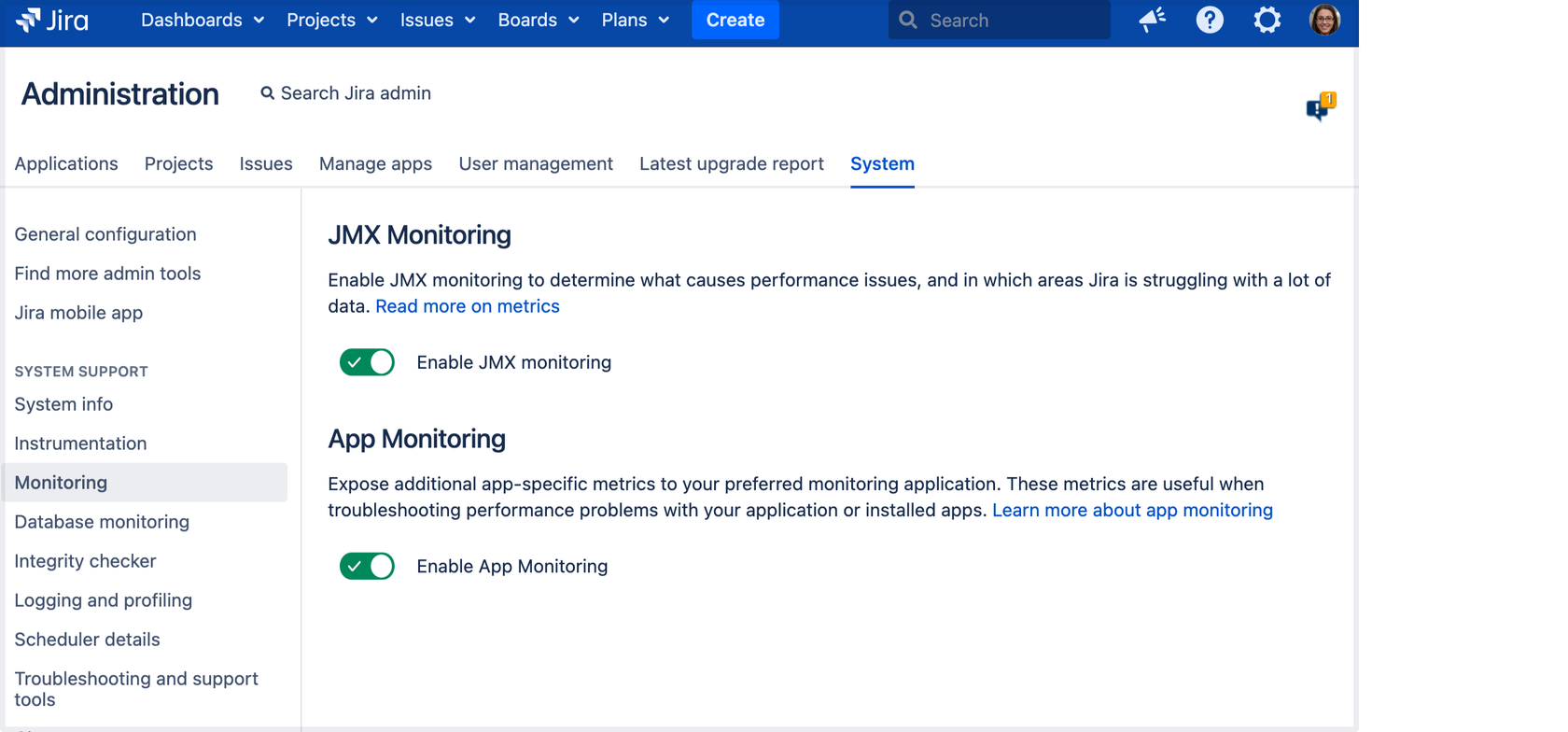**Caption:**

A detailed screenshot of a JIRA administration dashboard. 

The top navigation bar, set against a blue background, includes the following options: JIRA, Dashboards, Projects, Issues, Boards, Plans, and Create. Adjacent to these options are a search bar, notifications icon, a question mark for Help/Settings, and a profile picture. 

The main content area of the page features a white background with black text. Prominently, it displays numerous categories including Administration, Search, JIRA Admin, Applications, Projects, Issues, Manage Apps, User Management, Latest Upgrade Report, and System. 

Highlighted in blue, the section for JMX Monitoring offers a description: "Enable JMX monitoring to determine what causes performance issues and in which areas JIRA is struggling with a lot of data. Read more on metrics." Below this, an Enable JMX Monitoring toggle is visible.

Additionally, there's a segment on App Monitoring which explains: "Expose additional app-specific metrics to your preferred monitoring application. These metrics are useful in troubleshooting performance problems with your application or installed apps. Learn more about app monitoring," followed by another toggle switch.

Further down, the System Configuration section lists more administrative tools such as: JIRA Mobile App, System Support, System Info, Instrumentation, Monitoring (highlighted), Database Monitoring, Integrity Checker, Logging and Profiling, Scheduler Details, and Troubleshooting and Support Tools.

The screenshot aims to assist JIRA administrators in navigating various monitoring and configuration options to troubleshoot and enhance system performance.

Have a great day!